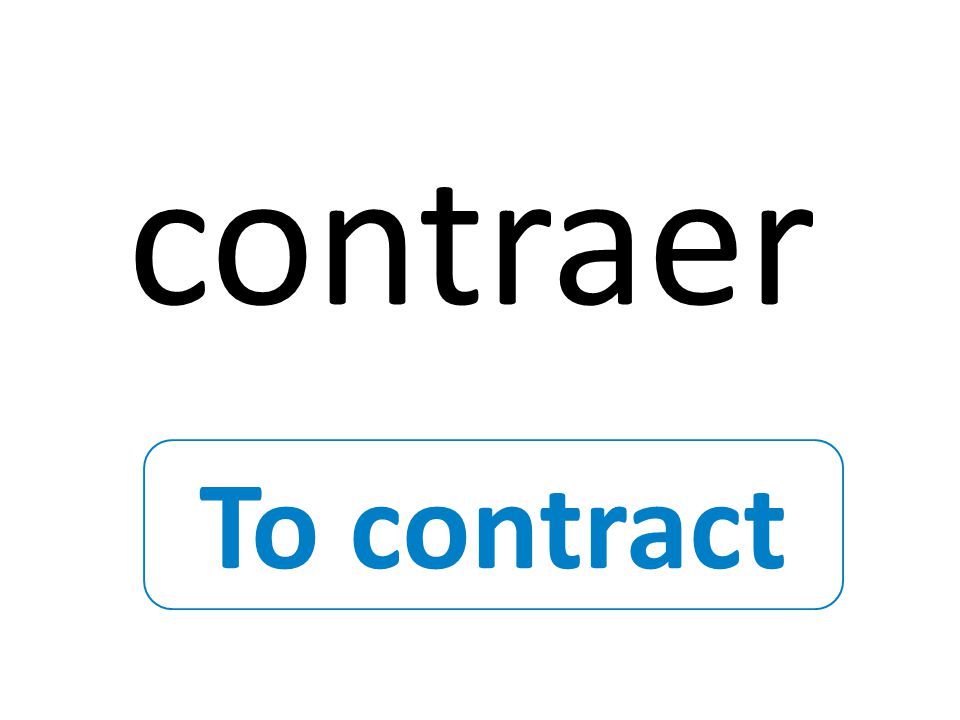The image features a simple white background displaying two distinct text elements. At the top, "Contraer" is written in black, all lowercase, and appears in a bold, typewriter-like font. Below it, a rounded rectangular border in light blue encloses the phrase "To contract." The word "To" is capitalized followed by the word "contract" in lowercase, both in black font. The blue-bordered rectangle is thin with slightly curved corners, framing the text with a modest amount of white space on either side.